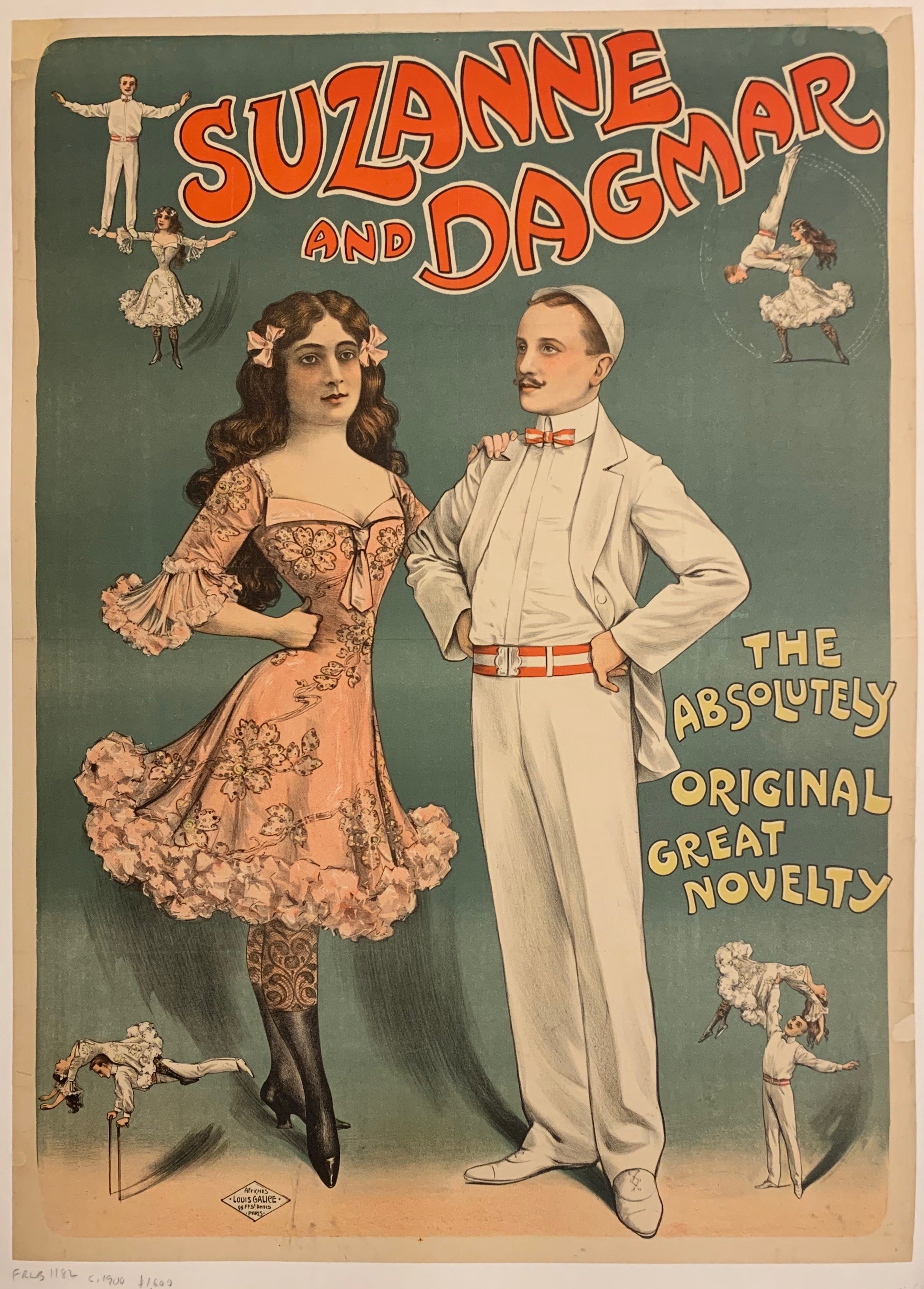This vintage-looking advertisement poster exudes the charm and nostalgia of old-time circus and carnival attractions. The hand-drawn artwork showcases two central figures, a woman and a man, surrounded by smaller illustrations of their acrobatic feats. The background is a grayish-teal color, giving the poster a sense of age with its yellowed paper accents from natural deterioration.

At the very top in large, funky orange text with a black and white outline, it reads "Suzanne and Dagmar." Below it features the tagline "The absolutely original great novelty" in yellow text on the bottom right corner.

The woman, referred to as Suzanne, has white skin and long, voluminous brown wavy hair adorned with pink bows on each side. She wears a knee-length, pink, flowery dress with a frilly bottom, complemented by flower-patterned stockings and tall black boots with heels. The man, Dagmar, also has white skin and is dressed immaculately in a white suit, complete with a white hat, shirt, slacks, and shoes. A striking red and white striped bow tie and matching belt add vibrant contrast to his outfit. He sports a handlebar mustache and stands confidently with his hands on his hips.

In each corner of the poster, smaller illustrations depict the duo performing various athletic acts: Dagmar balancing on Suzanne’s outstretched arm, Suzanne swinging Dagmar in a vertical circle, Dagmar balancing on canes while Suzanne lays on his back, and Dagmar lifting Suzanne overhead with one arm. These dynamic images contribute to the lively and captivating essence of the poster, making it a glimpse into a bygone era of circus excitement.